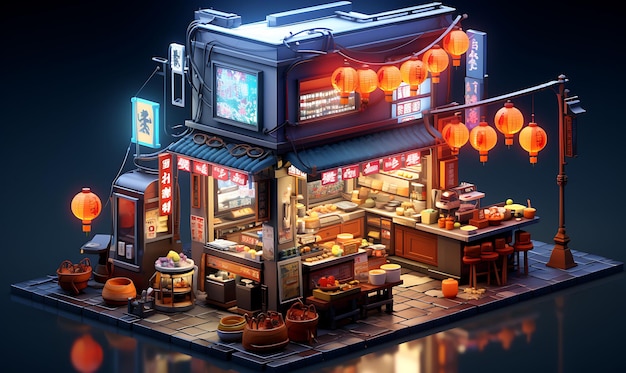This image appears to be a detailed, possibly AI-generated, isometric rendering of a small, futuristic, Asian-themed bakery or corner store in an urban setting. The shop, which has the appearance of a miniature model, is built on a brick and cobblestone-type base. The storefront is adorned with a mix of traditional and modern elements, featuring a blue and yellow awning with red flags.

The shop's façade includes glowing yellow balloons hanging from light posts and the building itself, while red signage with white font is prominently displayed, potentially indicating the type of goods or food available inside. The second floor showcases additional neon signs and Chinese lanterns, enhancing the store's vibrant, sci-fi aesthetic.

Inside, the open-concept store displays an array of bread, spices, and various goods on shelves and counters. There's a counter with stools on the right, along with baskets of goods around the corner and a vending machine to the left. Seating is available on the perimeter of the shop and there are plates set on a table near the left entrance.

The detailed rendering captures reflections from the lighting and Chinese lanterns on the slate gray stone sidewalk, contributing to the realistic though clearly artificial composition of the scene.